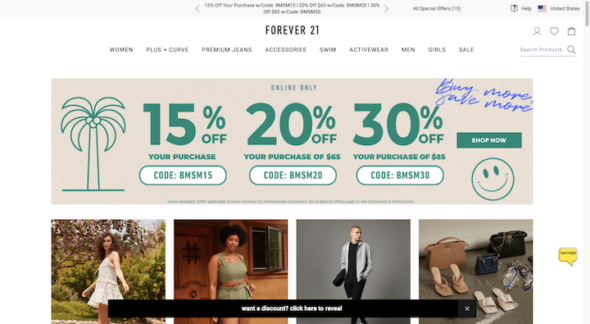This horizontal rectangular image depicts the homepage of the Forever 21 website. The page opens with the "Forever 21" brand name prominently displayed at the top center in bold black font, where "21" is written numerically. Just below this, spanning from left to right, are various category tabs in all capital letters and black font: WOMEN, PLUS, CURVE, PREMIUM JEANS, ACCESSORIES, SWIM, ACTIVEWEAR, MEN, GIRLS, and SALE. 

Beneath the navigation bar is a horizontal beige banner featuring a promotion. On the left-hand side of this banner is an icon of a palm tree. Bold green numbers declare "15% OFF" with the percentage sign, and directly beneath this, in bold green capital letters, is the phrase "YOUR PURCHASE." A white oval with a green border underneath contains the word "CODE" in green capitals, followed by a placeholder for the promotional code. 

To the right of this, additional discounts are shown: "20% OFF" for purchases over $65, and "30% OFF" for purchases over $85, each similarly styled with codes beneath. 

In the upper right corner of the beige banner, the phrase "BUY MORE, SAVE MORE" is written in blue script, with "SAVE MORE" positioned below "BUY MORE." Adjacent to the discount listings is a green horizontal rectangular button with the phrase "SHOP NOW" in white capital letters. Beneath this button is a smiley face with green eyes, a green smile, and a green outline.

Centered at the top of this tan promotional image, above the discount details, it states "ONLINE ONLY." Below this statement, there is a small white section followed by four vertical rectangular images. The first two images showcase women modeling various outfits, the third features a man, and the fourth displays three different pocketbooks with matching shoes arranged in front. 

At the very bottom of the page, a horizontal rectangular banner in white font reads, "WANT A DISCOUNT? CLICK HERE TO REVEAL," providing an enticing call-to-action for additional savings.